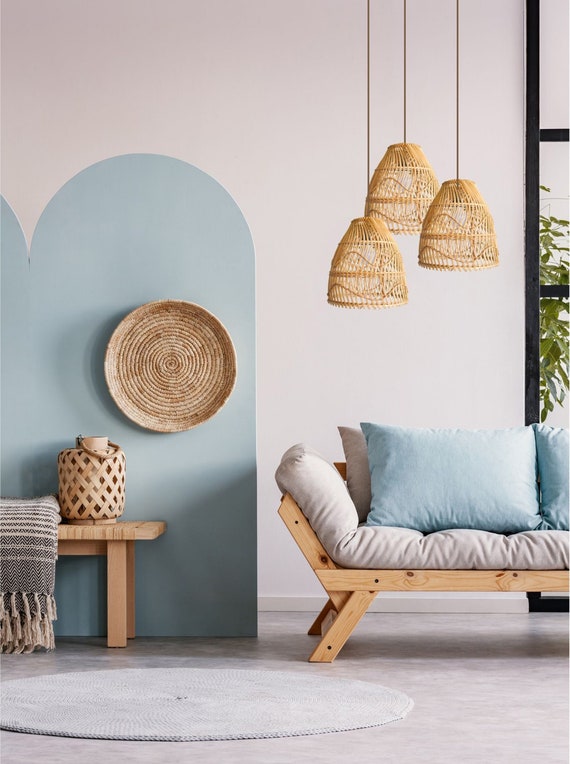This vertical image showcases a modern, beautifully designed living room scene with a calming blue and white color theme. The background features a white wall with an archway shape painted in light blue, accentuated by a round wicker basket hanging in the center. To the left, a light blue dressing screen with a woven basket hanging from it stands out. In front of this, a natural wood table displays another wicker basket with a handle and a neatly draped gray and tan blanket. The floor is white, complemented by a circular white rug on the left side of the scene. In the mid-ground on the right, a wooden-framed loveseat with a white cushion is adorned with light teal and sky blue pillows. Above, three wicker lamps hang from the ceiling, adding texture and warmth. A floor-to-ceiling window on the right edge reveals a glimpse of greenery outside, enhancing the scenic and serene atmosphere of the space.